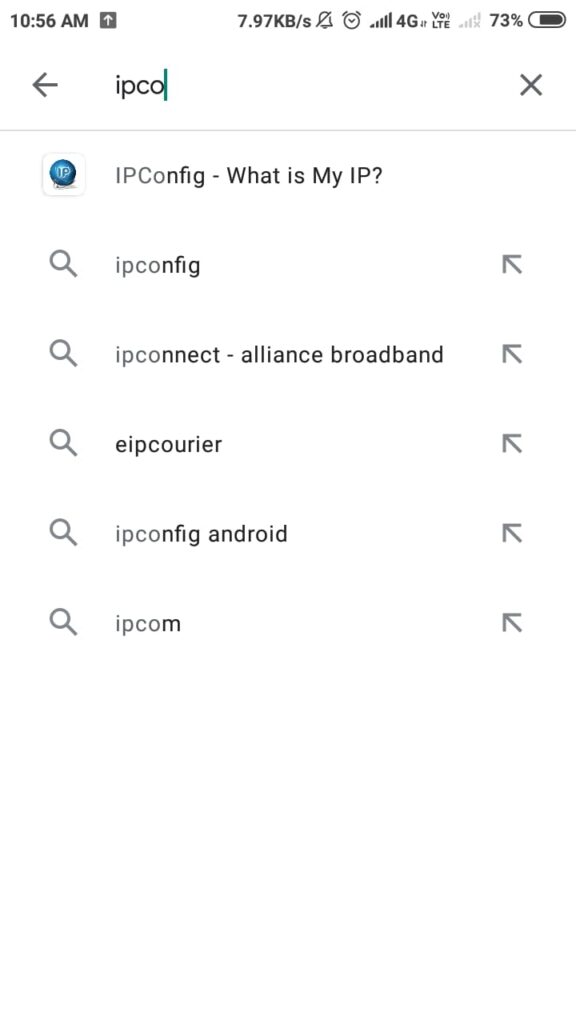A screenshot of a mobile search page taken at 10:56 AM displays a clean interface with a white background. At the top, centered, lies a search bar where "IPCO" has been typed. To the left of the search bar, there's a left-pointing arrow, and to the right, an 'X' icon. Below the search bar, a list of search results is visible, including options like "IPConfig," "What is my IP," "IPConfig," "IPConnect," "Alliance," "Broadband," "EIP," "Courier," "IPConfig," "Android," and "IPCOM." Each search result is accompanied by a magnifying glass icon to the left and a diagonal arrow pointing up to the left on the right side. Across the middle of the image, partially cropped out, is a grey text watermark reading "Termark" or "Watermark." Further below, additional grey text states "this image is protected."